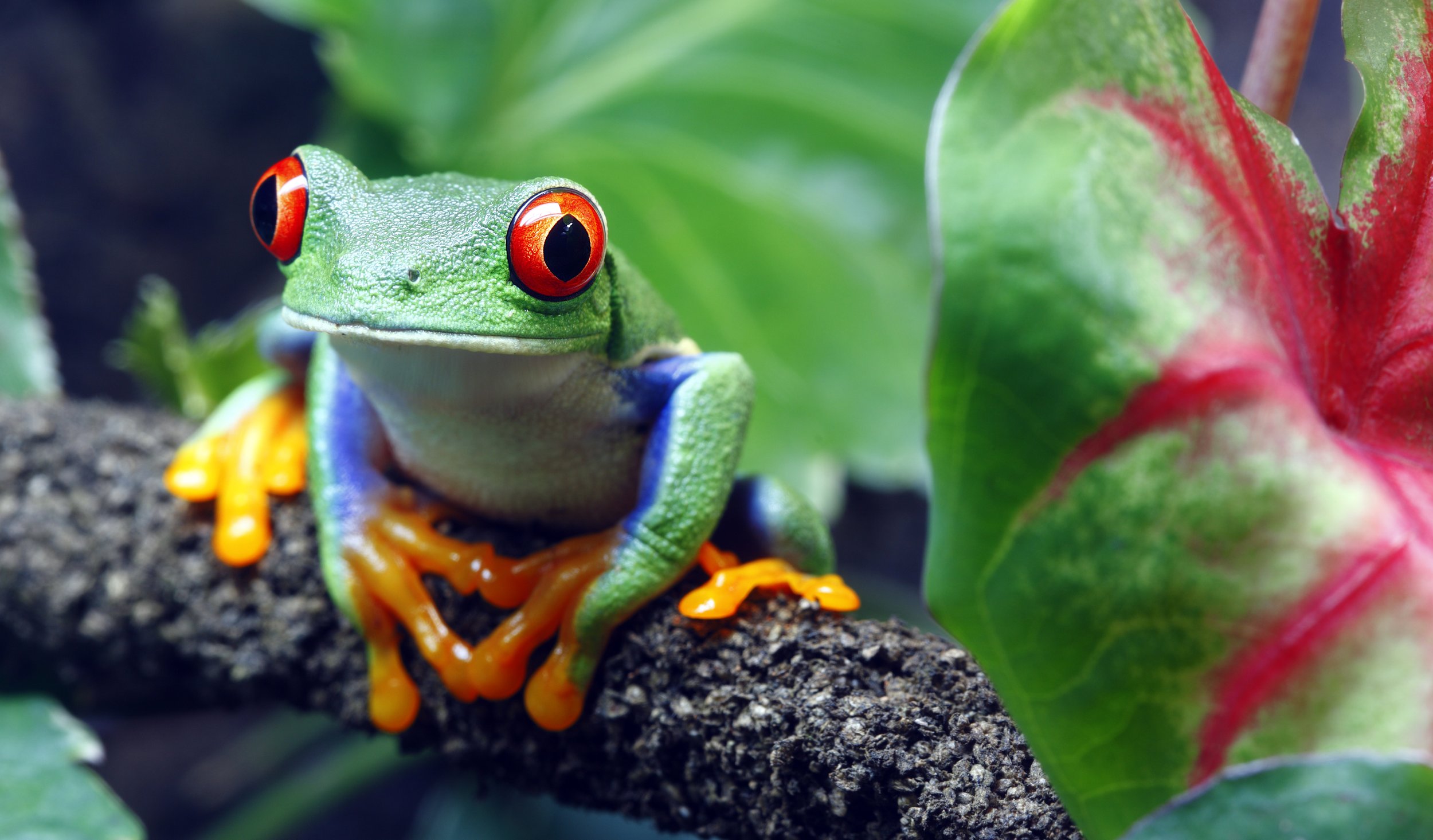A vibrant and detailed close-up photograph of a brightly colored tree frog perched on a dark charcoal gray branch amidst lush rainforest vegetation. The frog, positioned on the middle left side of the photo, showcases striking features: large, wide-open red eyes with black pupils, a light green back, and a white underbelly and lip. Its neon orange three-pronged fingers and feet stand out vividly against its brilliantly blue inner arms. The frog's arms have a unique pattern with a white line running up their length. The surroundings exhibit a variety of textures and colors, with prominent leaves in shades of forest green and hints of red at their centers, adding to the vivid jungle scenery. The tree frog, seemingly alert and possibly poisonous due to its bright coloration, is an eye-catching centerpiece in this rich tableau of natural beauty.